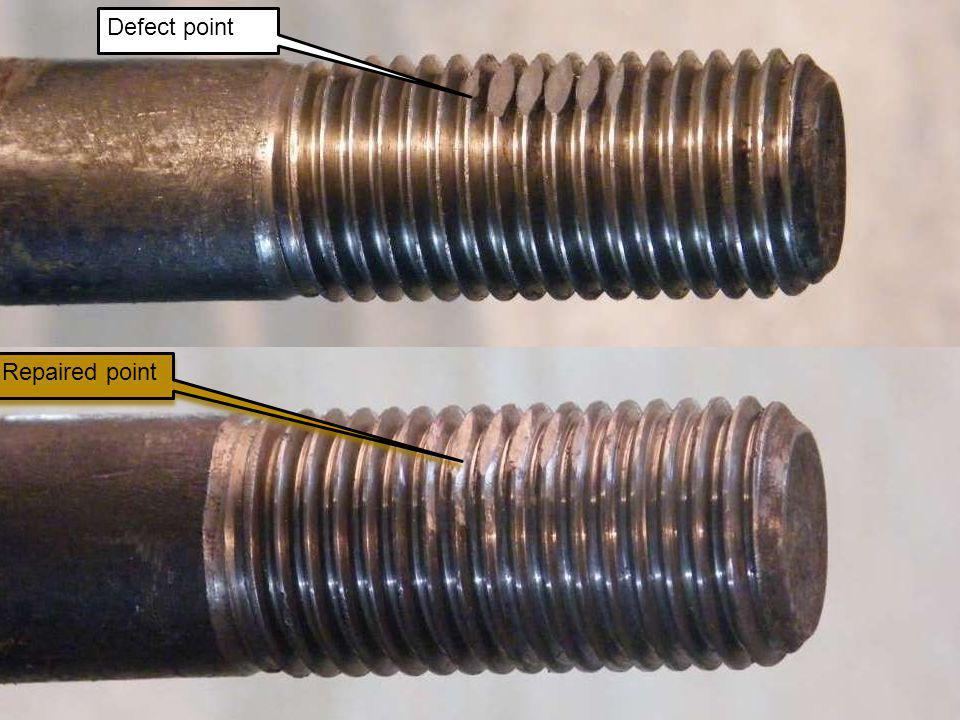The image features a detailed before-and-after comparison of two bolts against a blurred and abstract background. The top half shows a close-up of a defective bolt with a bronzed, silverish metallic hue. This bolt has flat divots where it should have grooved edges, a defect highlighted by a white text box outlined in black, labeled "defect point." In contrast, the bottom half of the image presents the same bolt after repair. The once-defective areas now appear smooth and polished, resembling a standard, functional bolt. This repaired bolt is indicated by a yellow text box, also outlined in black, labeled "repaired point." Both bolts are aligned parallel to each other, emphasizing the transformation from defective to repaired. The text colors and contrasting backgrounds further accentuate the differences between the two states of the bolt.